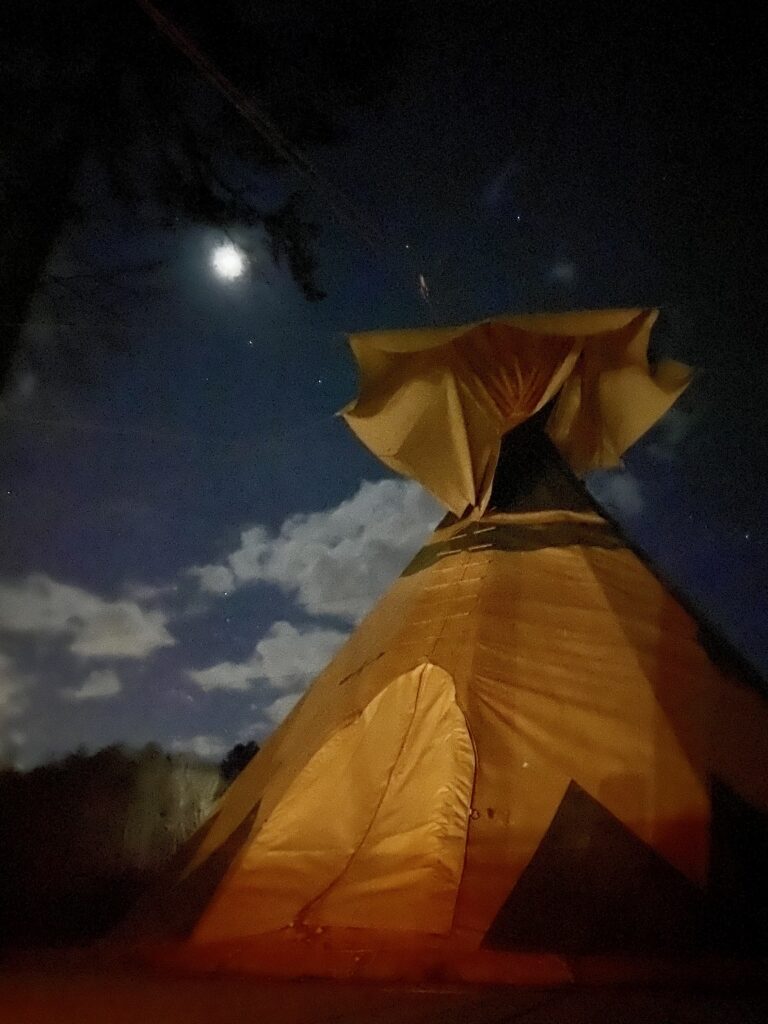This nighttime photograph captures a rustic teepee set against a dark, cloud-filled sky. The teepee, predominantly a light tan color, stands tall on the right-hand side of the image, its triangular shape accentuated by an arch-shaped door and various triangle decorations near the base. Crowning the structure is a light tan flap resembling a floral shape. Above the teepee, power lines or similar wires stretch across the night sky, where a bright, white moon shines through scattered gray clouds. To the left, the upper branches of a tree are visible, further emphasizing the natural surroundings. The ground below is dimly illuminated, hinting at a hilly landscape in the background along with more distant trees.